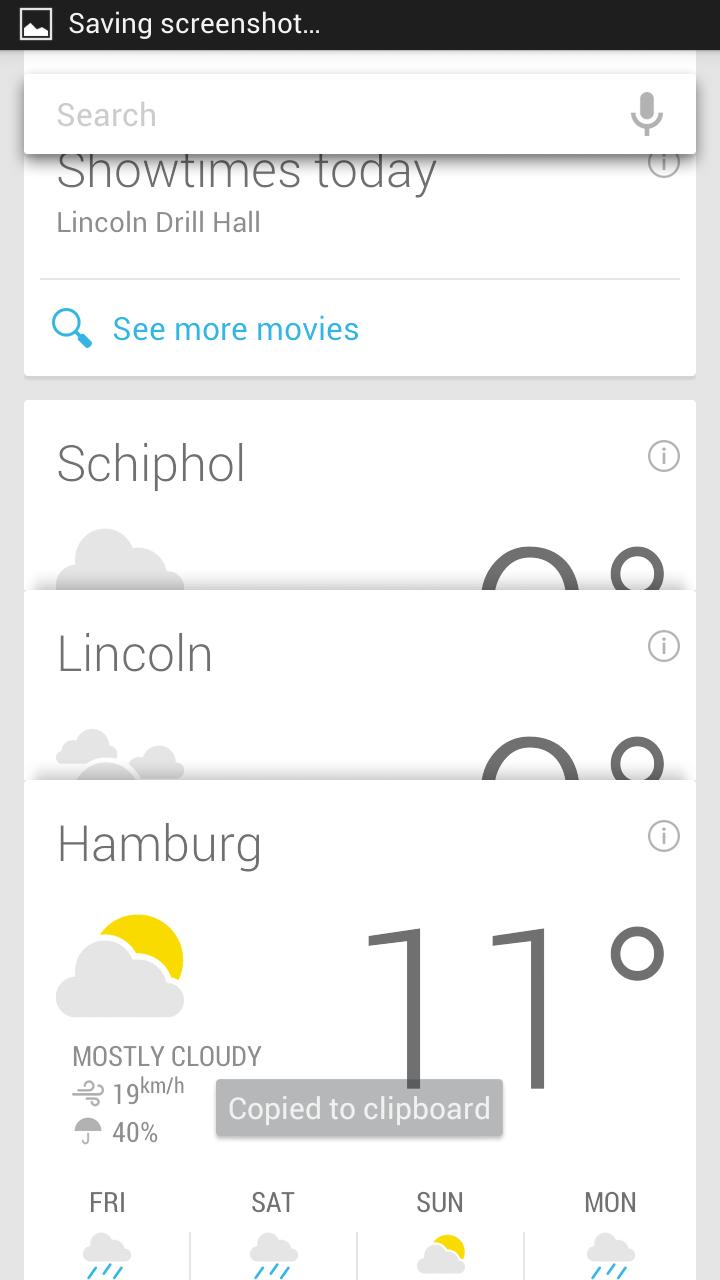A mobile phone screenshot captured while using a multi-functional app that combines weather forecasting with entertainment listings. The app interface is displayed on a white background and features card-style elements for different cities and showtimes. 

At the top of the screen, a section titled "Showtimes Today at Lincoln Drill Hall" is visible, along with an option to "see more movies." Just below, weather information is presented for various cities:
- **Schiphol** (partially cut off): Weather details are incomplete.
- **Lincoln**: Display shows clouds, but the temperature is either cut off or set to zero.
- **Hamburg**: Illustrated with a cloud and partial sun, indicating mostly cloudy weather with a temperature of 11 degrees (unit unspecified). Additional details mention a wind speed of 19 km/h and a 40% chance of precipitation, depicted by an umbrella icon.

Further down, a forecast summary suggests that the weather for Friday, Saturday, Sunday, and Monday is expected to be rainy, aligning with the format used for Hamburg. 

At the top right corner, a search box accompanied by a traditional microphone icon is present, indicating voice search functionality. The phrase "saving screenshot" appears in the notification area, symbolized by a small picture frame icon on a black background.

Overall, the app appears to be a hybrid platform potentially utilized for both checking weather updates and finding local movie showtimes, offering a seamless user experience with its card-like interactive design.